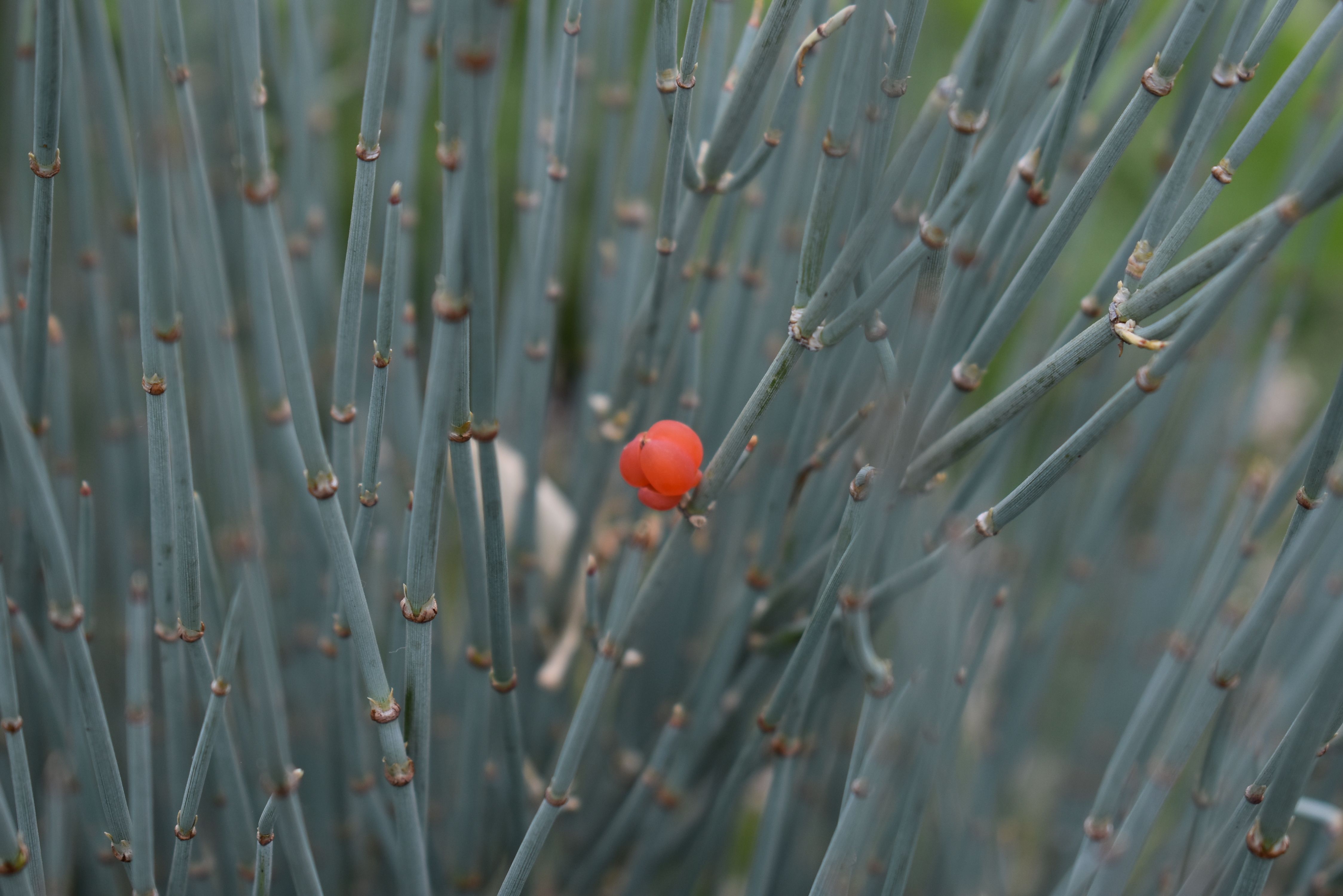This outdoor image is a close-up of a small bush-like plant with slender, segmented stems resembling miniature bamboo. The branches are yellowish to grayish-green and feature periodic brown, knuckle-like joints. One distinctive branch in the center, leaning slightly to the right, showcases a budding, reddish-orange flower or fruit emerging from one of these joints. The flower appears pillowy and bulbous, hinting at the early stages of growth. Surrounding the plant is a background blurred and out of focus, with green leaves and a soil bed visible, indicating a springtime setting. The overall lighting is muted, suggesting the photo was taken on a cloudy or overcast day.